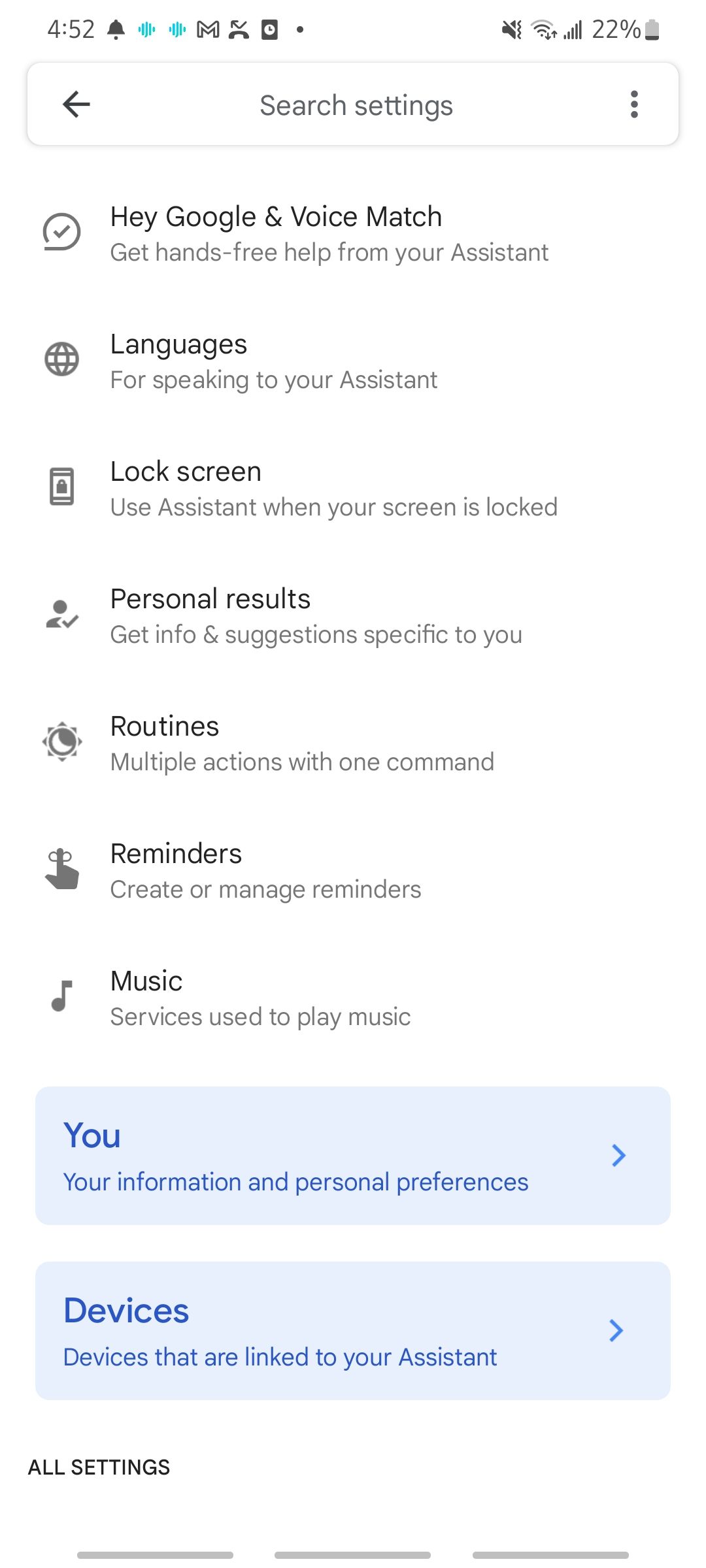The image displays a detailed screen from a mobile device, showcasing the Google Assistant settings interface. Here's a breakdown of the elements present in the image:

At the top:
- A bell icon, likely a notification.
- An unspecified item or icon.
- The Gmail app icon.
- A handset icon probably representing a call function.
- An arrow, indicative of navigation (possibly a back arrow).
- A "Done" button.
- A speaker icon that is currently not enabled.
- Wi-Fi icon indicating connection status.
- Full signal bars showing strong network reception.
- Battery status at 22%.

Main screen details:
- A left-facing arrow indicating back navigation.
- A search bar labeled "Search settings."
- An ellipsis (dot, dot, dot) for accessing more options.
- Various settings for Google Assistant:

   1. **Check mark** - to select or confirm.
   2. **"Hey Google" Voice Match** - Options for hands-free assistance.
   3. **Languages** - Choices for communicating with the Assistant.
   4. **Lock screen** - Control over using the Assistant with the screen locked.
   5. **Personal results** - Enabling personalized information.
   6. **Routines** - Setting up multiple actions triggered by a single command.
   7. **Reminders** - Options for creating or managing reminders.
   8. **Music** - Configuring services for music playback.
   9. **Information** - General informational settings.

Background details:
- The top of the screen has a blue background.
- A red arrow, probably marking significant settings or alerts.
- A section labeled "Devices" listing devices linked to the Assistant.
- A right-facing arrow next to each option for further details.

Bottom of the screen:
- Below the main settings, there is an "All settings" option.
- Separating elements are grey lines against a white background.

This comprehensive description captures the detailed elements and functionality displayed on the screen for better understanding.